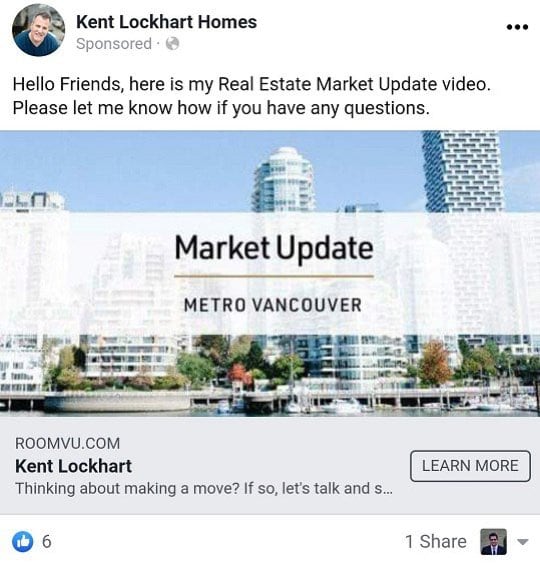In the upper left corner of the image, there's a circular profile picture featuring a light-skinned man with brown hair, smiling while wearing a blue sweater. Beside this profile picture, black text reads "Kent Lockhart Homes" followed by the word "Sponsored" and an image of Earth. The message beside it states, "Hello, friends. Here is my real estate market update video. Please let me know if you have any questions."

The background of the image displays a large cityscape with tall buildings and boats in a marina-like area. Beneath this background, there is underlined text that reads "Market Update" and below that, "Metro Vancouver" in black text. 

In the lower left corner, "RoomVu.com" is written, followed by Kent Lockhart's name again. The text reads, "Thinking about making a move? If so, let's talk," accompanied by a square button with "Learn More" written inside it. There is also an indication of one share, with an accompanying square profile picture of a man wearing a suit and having short hair.

On the left side of the image, there is a blue circle with a thumbs up sign inside it, alongside the number six, representing six likes on Facebook.